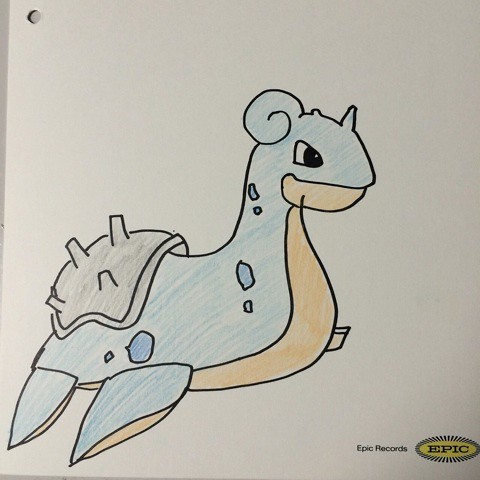This illustration, rendered in vibrant crayon or colored pencil, is presented on a white sheet of paper with a small hole punctured in the top left corner. In the bottom right corner, the words "Epic Records" are inscribed, with "Epic" prominently displayed within an oval emblem. Dominating the center of the image is a whimsical sea creature, vividly depicted with a dual-toned body: tan on the underside and a rich blue on top, mottled with distinctive spots. The creature features two fins on its right side and bears a menacing shell or saddle adorned with prominent spikes jutting upwards from its back. Its head is crowned with a small horn, and a spiral-like structure encircles the rear of its head. The sea creature's expressive face showcases a visible side profile of its mouth, with the top being blue and the underside a sandy tan, completing the fantastical depiction.